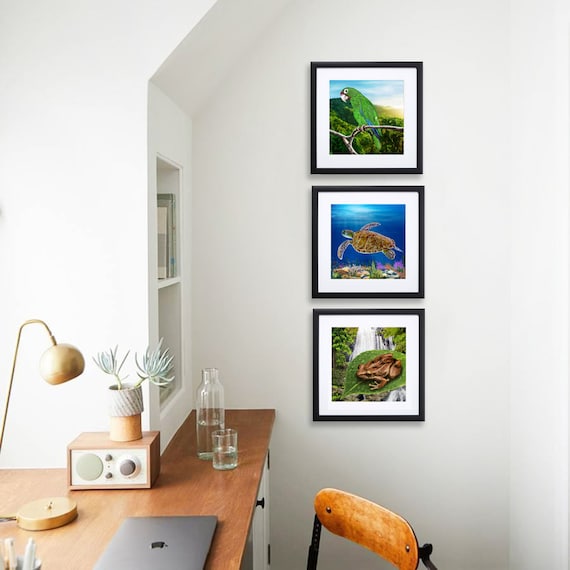In this photograph of a well-organized office space, the setting features a minimalist design with white walls adorned by three black-framed pictures. The first frame showcases a vibrantly colored green parrot amongst lush green foliage. The second frame captures a serene scene of a brown sea turtle swimming effortlessly in the ocean. The last frame presents a close-up of a brown frog perched on a green leaf.

Beneath the artwork, a contemporary, black-framed chair with an oval-shaped, light wooden backrest is prominently positioned. Adjacent to this, a pristine white cabinet serves as the base for a light-brown wooden desktop, creating a harmonious blend of colors and textures.

On the desktop, a few tasteful items are neatly arranged. A sleek, golden table lamp adds a warm touch, while a glass of water sits ready at hand. Completing the workspace setup is an Apple laptop, symbolizing productivity and modernity, accompanied by what appears to be a compact radio and a few decorative items, adding a touch of personal flair to this inviting office environment.